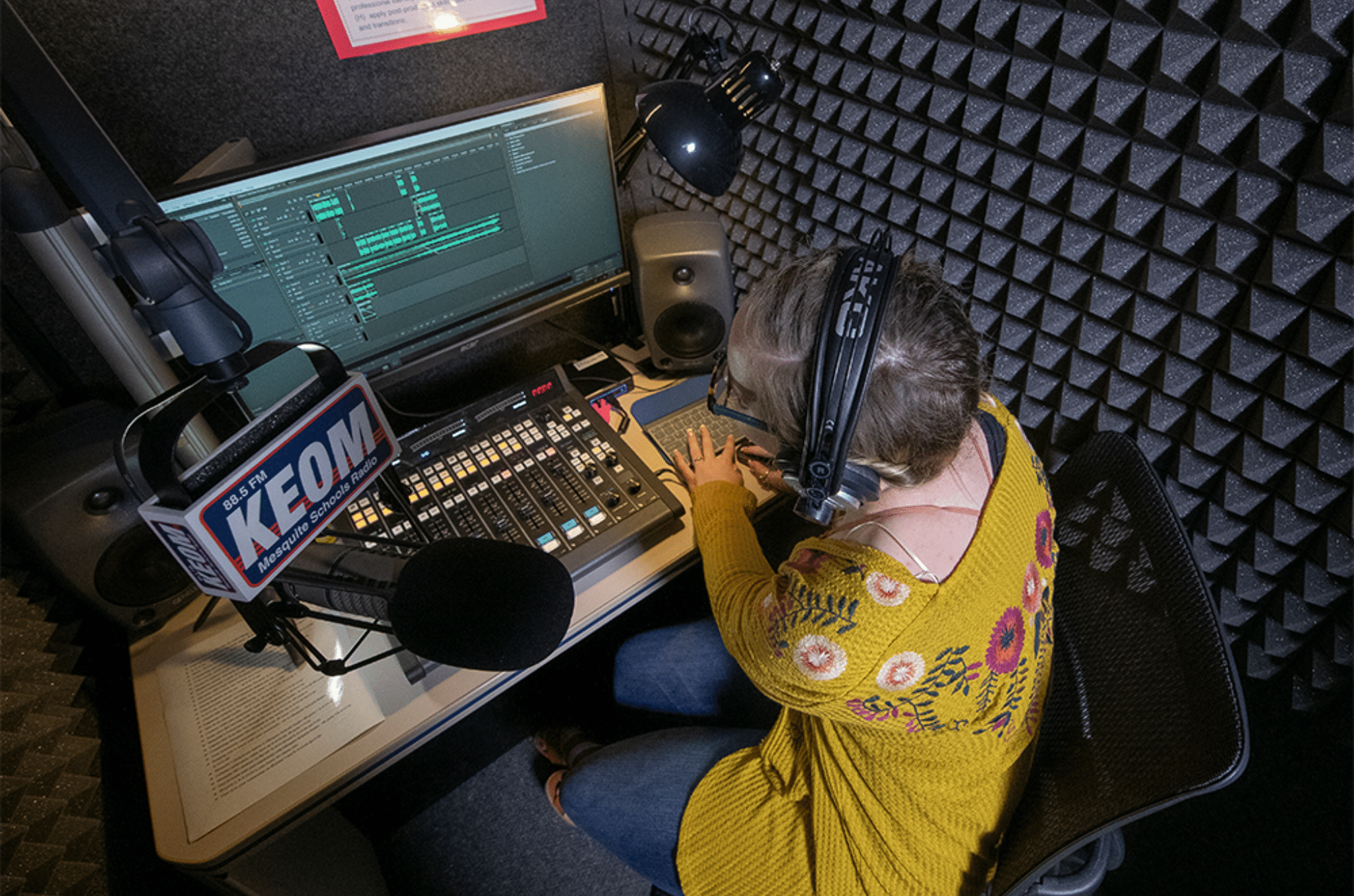The photograph, shot from overhead in a soundproof recording studio, captures a female radio DJ for 88.5 FM KEOM Mesquite School Radio. The studio features soundproof foam on the walls, a prominently displayed microphone labeled "KEOM 88.5 FM Mesquite School Radio," and an array of equipment including a soundboard, speakers, and a keyboard. The DJ, identifiable by her black AKG headphones, short hair, and glasses, is wearing a bright yellow floral blouse and blue jeans. She sits in a chair, concentrating on a monitor with green bars, her hands actively using a mouse while she manages the equipment on her desk, which also includes a desk lamp.